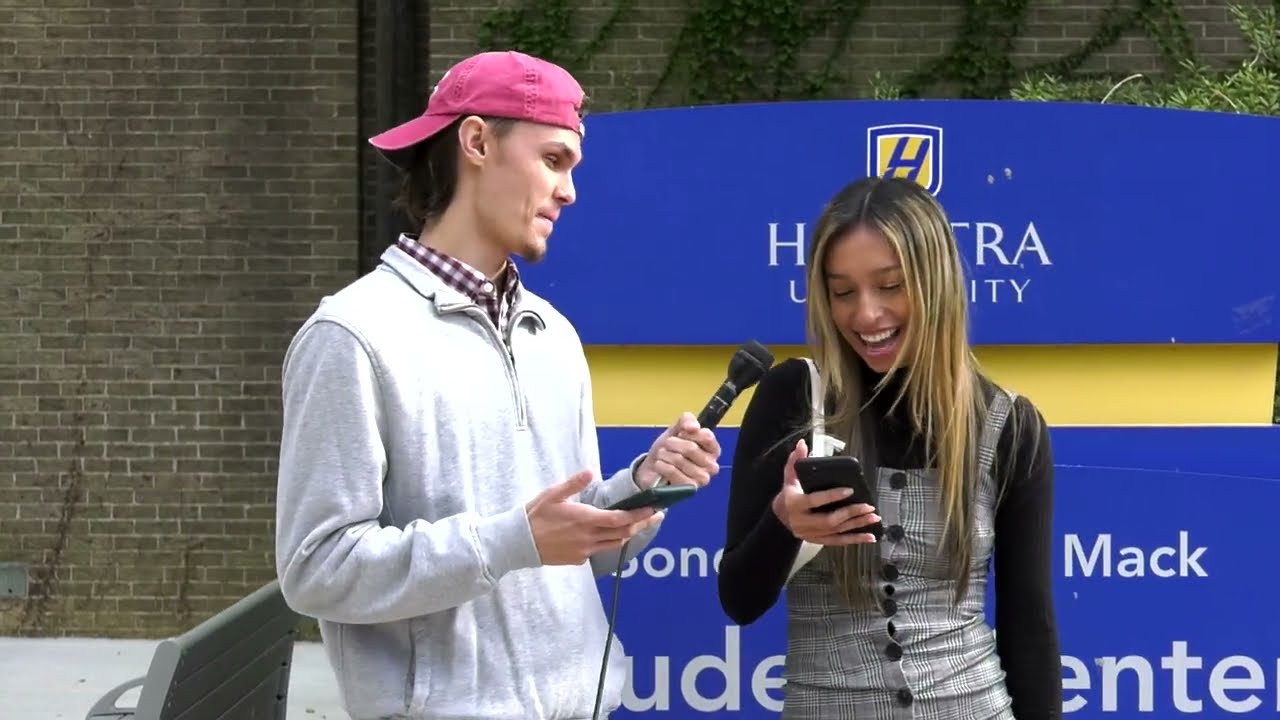In the image, two young people are standing in front of a Hofstra University sign. The man on the left has long black hair and is wearing a backward red hat, a light gray zip-up sweater with a red and white plaid collared shirt underneath. He is holding a black microphone in one hand and a black phone in the other, seemingly interviewing the woman next to him. She has blonde hair with dark roots, suggesting dyed hair, and is smiling while looking at her black phone. She is wearing a black long sleeve undershirt and a checkered black and white dress with big black buttons. They are standing in front of a large blue and yellow sign that partially reads "Hofstra University" and "Student Center," with the rest obscured by their positions. Behind them is a grayish brown brick wall with ivy growing on it, and to the left of the man is a brown wooden bench with metal railings. The scene appears to be outside on the university campus.